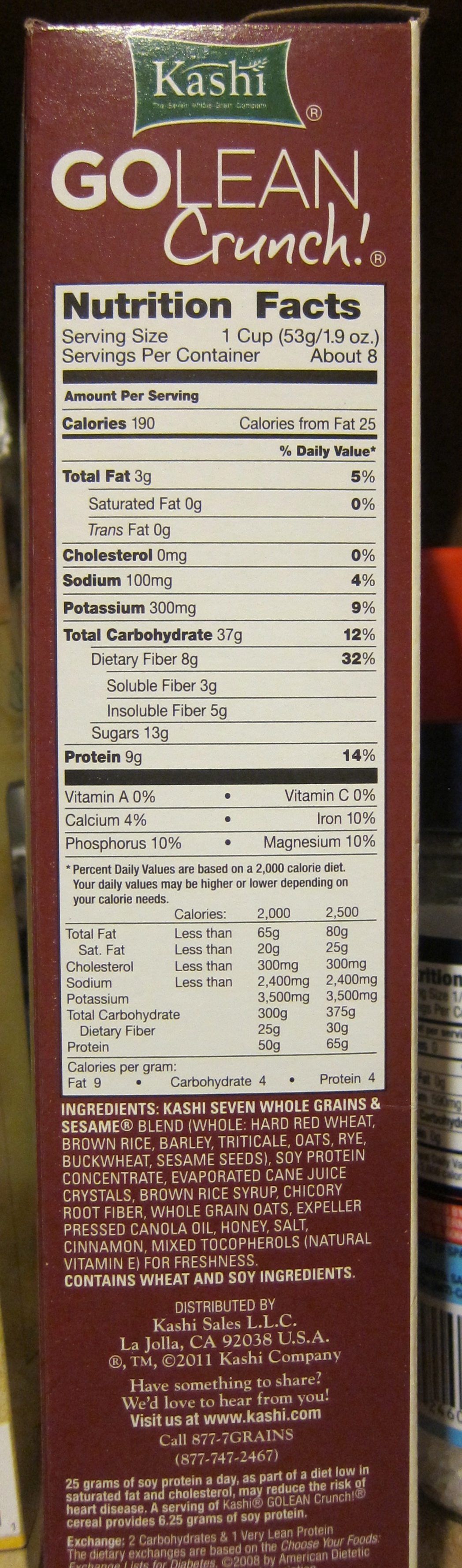This color image is a vertically-oriented snapshot showcasing the side of a Kashi product box, specifically the "Go Lean Crunch." The box itself is a rich brown color. Prominently displayed at the top is the Kashi logo, rendered in green with white lettering. Directly below the logo, "Go Lean Crunch" is written in bold white letters. This is followed by a comprehensive list of nutritional facts, detailing the health benefits of the product. Further down, the ingredients are meticulously listed. The distributor’s information is also provided, identifying La Jolla, California, as the location, along with a contact phone number for customer inquiries. There are two additional, smaller blocks of text that remain illegible. The photograph appears to have been taken inside a cupboard, as suggested by the visible edge of another product's nutritional label in the lower right-hand corner of the image.